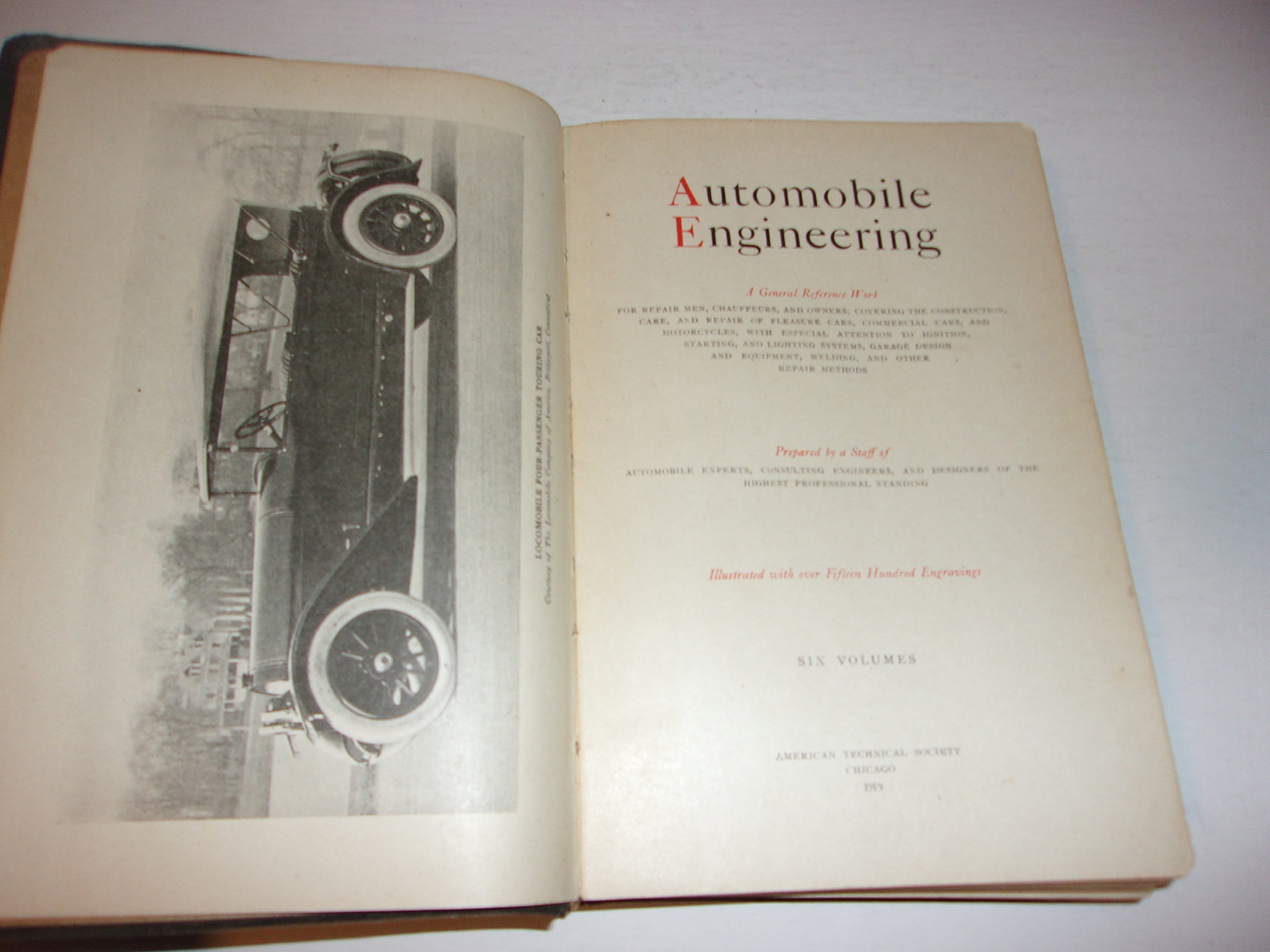This detailed close-up photograph captures an old, weathered book opened to the first page, resting on a white table. The left page prominently features a vertical photograph of a black, classic car, likely a Ford Model T, with distinctive white wheels. The car is oriented such that the front is at the bottom of the page, and the back is at the top. On the right, the text "Automobile Engineering: A General Reference Work" is displayed, with "A" and "E" in red ink. Below this, it reads "Prepared by a Staff of," followed by additional text that is partially obscured. Further down, it mentions "Illustrated with 1500 Engravings" and indicates that the work is comprised of "Six Volumes." The publisher, "American Technical Society, Chicago," is noted at the bottom, along with a faint and hard-to-discern number that might be "1889." The pages appear faded and aged, indicative of the book's antiquity.